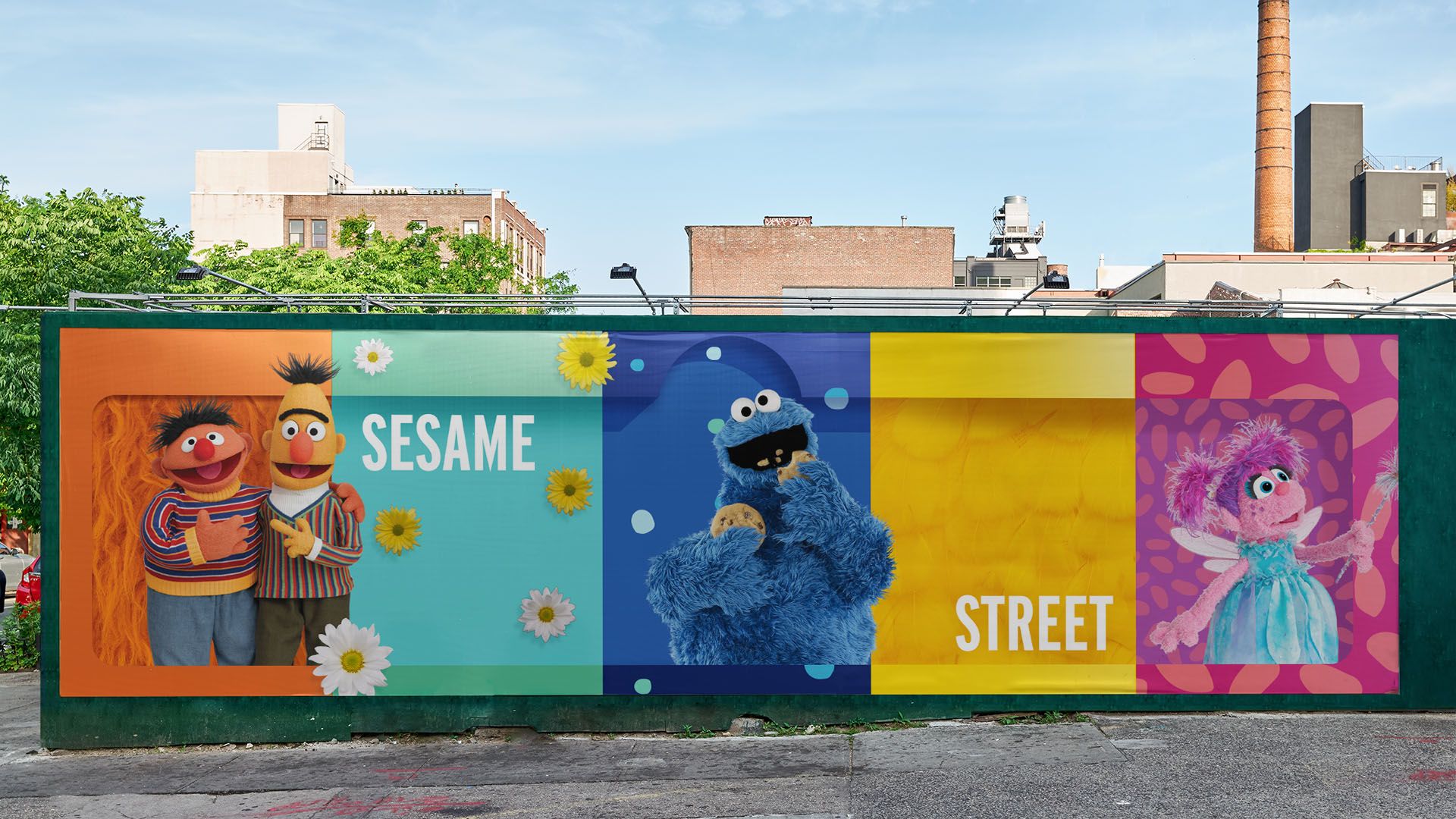The photograph captures a vibrant city street on a bright, sunny day. Dominating the scene is a colorful billboard against a backdrop of towering buildings, green trees, and a clear blue sky dotted with fluffy white clouds. The billboard promotes the beloved PBS children's show Sesame Street and consists of five distinct, eye-catching panels framed by a green border.

On the far left, the orange-colored panel features the iconic duo, Bert and Ernie. Ernie, with his orange skin, red nose, and black hair, is dressed in a horizontally striped orange and red shirt with blue pants. Bert, sporting a longer face, orange nose, and vertically striped shirt, points at Ernie, creating a lively interaction. Both are set against a backdrop of a brown fence.

Next to them, the light blue panel bears the word "Sesame" and is adorned with yellow and white flowers. The following dark blue panel depicts Cookie Monster eagerly devouring a cookie, his bright blue fur contrasting with the blue polka-dotted background.

The fourth panel is yellow and simply states "Street," balancing the composition. The final panel on the far right features a whimsical portrayal of a new Sesame Street character, a fairy princess with pink hair, pink face, and blue dress. She stands against a purple and pink floral background, looking upwards with small white wings and holding a wand.

The bustling city street scene, complete with lampposts, a graffiti-adorned wall, and paved sidewalks, adds to the dynamic setting, making the billboard an eye-catching and cheerful fixture in the urban landscape.